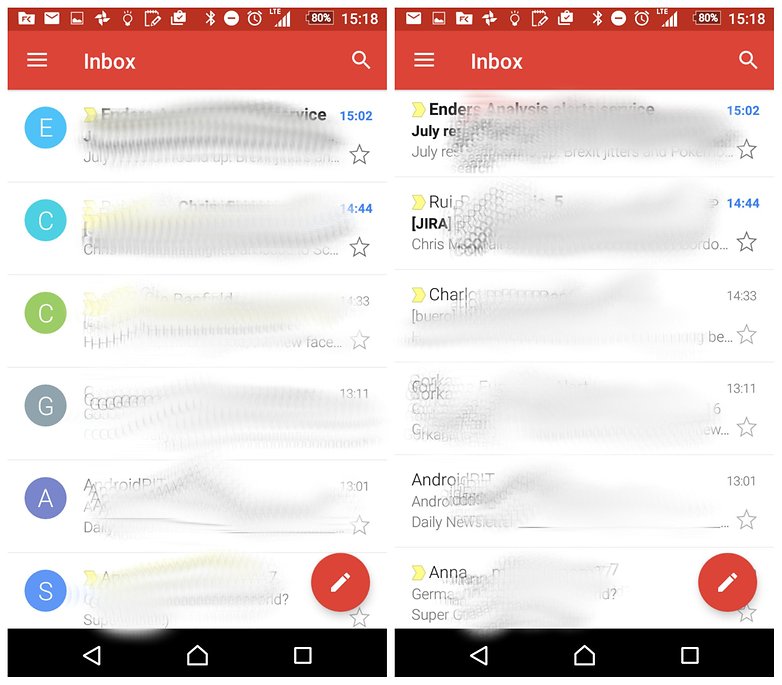The image features a white background with two distinct screens side by side, each presenting a variety of interface elements and icons.

**Left Screen:**
- The top portion contains a prominent red bar displaying a battery level at 80%. Numerous small icons span across the top, with the time indicated as 15:18. 
- Below this, the interface includes a magnifying glass icon for search functionality, flanked by three horizontal lines representing a menu and an 'Inbox' label.
- The main section of the screen shows several objects:
  - A large white circle with the letter 'E' inside, accompanied by the time 15:02 and a star symbol.
  - A blue circle containing the letter 'C', marked with the time 14:44 and a star.
  - A green circle with the letter 'C', paired with the time 14:33 and a star.
  - A grey circle showing the letter 'G', detailed with the time 13:11, where the star is greyed out or inactive.
  - A dark blue circle featuring the letter 'A', next to the time 13:01 and a star.
  - A blue circle hosting the letter 'S'.
- Located towards the bottom is a prominent red circle with a pencil icon in the center, accompanied by a star underneath. 
- At the very bottom, there's a black rectangle comprising icons of a triangle, a house, and a square.

**Right Screen:**
- Similar to the left screen, the top section has a red bar indicating an 80% battery level, small icons, and the time noted as 15:18.
- Icons for a menu, inbox, and a search magnifying glass are again displayed, with 'Inbox' labeled.
- This screen additionally features several items:
  - Each object on this screen is preceded by a yellow arrow pointing to the right.
  - Time stamps and star symbols are presented as follows: 15:02, 14:44, 14:33—all with star symbols.
  - A grey circle showcasing the letter 'G', marked 13:11 and a star.
  - An area with text resembling "Android", proceeded by times and stars, followed by the name "Anna" and potential German text stating "Super."
- As with the left screen, there is a large red circle with a pencil icon at the bottom right and a star positioned below it.
- The bottom interface is rounded off with the same black rectangular box containing a triangle, house, and square icons.

Both screens illustrate a meticulously designed user interface, filled with diverse and interactive elements highlighted by their distinct colors and symbols.